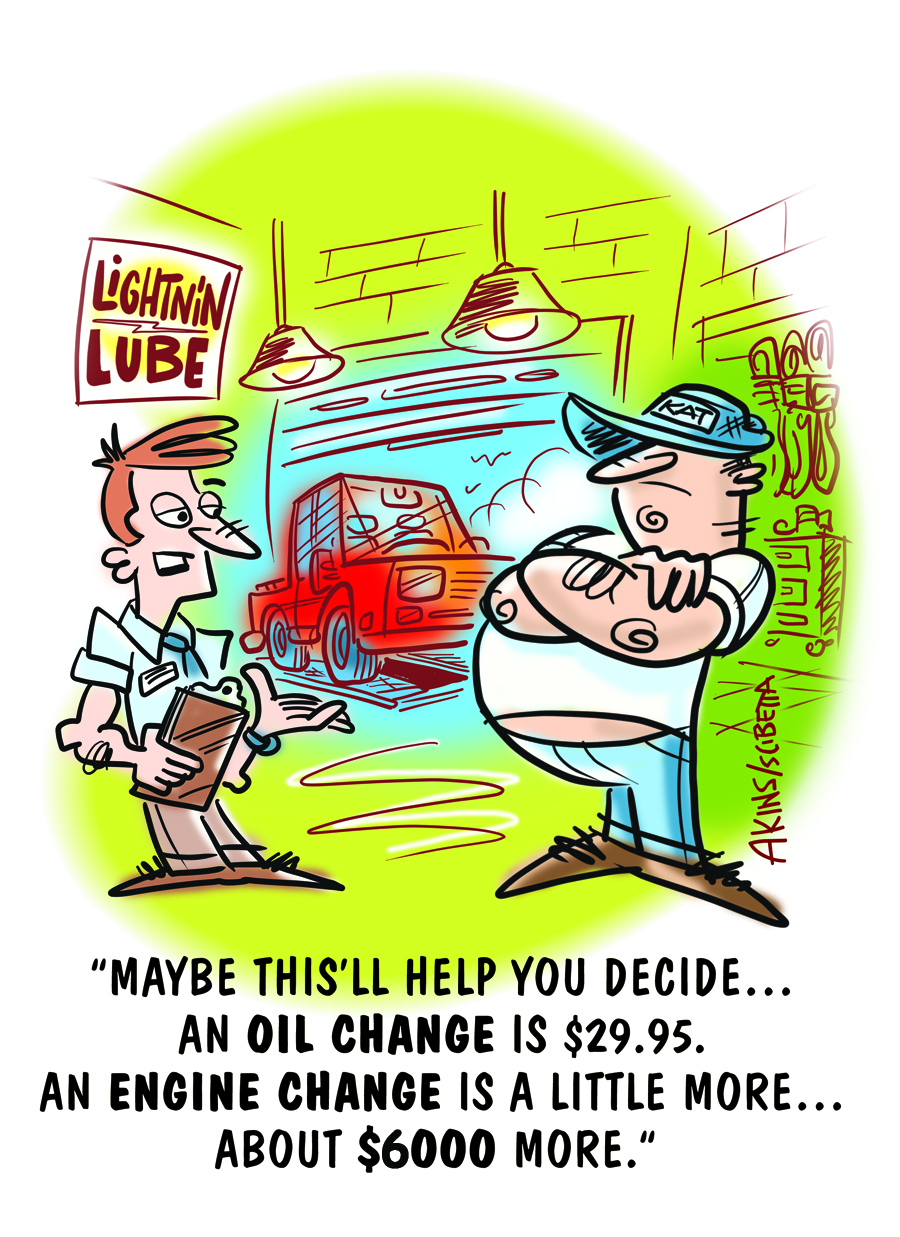In a colorful comic drawing with a green wall and ceiling, two men stand inside a garage, illuminated by two hanging lights with yellow bulbs. The left side displays a sign reading "Lightnin' Lube." The man on the left, holding a brown clipboard, has a sharp pointy nose and protruding eyes, and he wears a shirt and tie. He appears to be explaining something to the larger man on the right, who has his arms crossed, obscuring part of his blue baseball cap with "KAT" on it. This man wears a white short-sleeve t-shirt that doesn't quite cover his belly, paired with blue pants. In the background is a red car. At the bottom of the image, the text reads: "Maybe this will help you decide. An oil change is $29.95. An engine change is a little more, about $6,000 more."